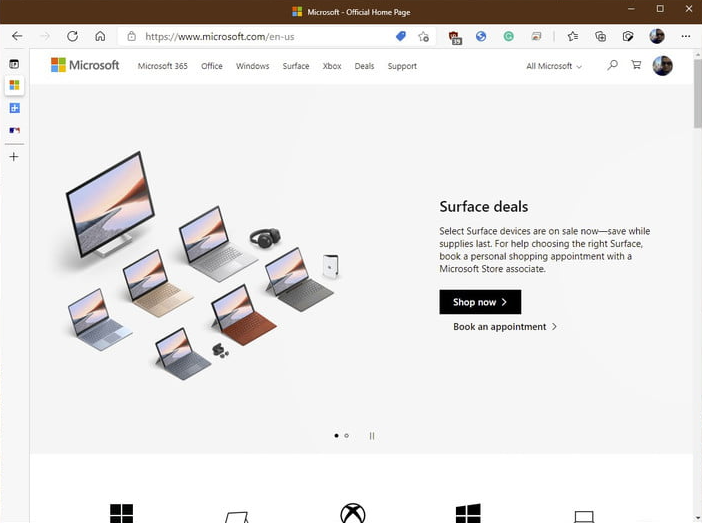The image depicts a screenshot of the official Microsoft homepage on a web browser, likely Google Chrome. The image itself is slightly wider than it is tall, approximately 20% wider. At the top of the image, there is a brown navigation bar that occupies about 5-10% of the image's height. Centered within this bar is the Microsoft logo in white, accompanied by the text "Microsoft - Official Homepage."

Beneath this navigation bar are typical web browser elements, such as tabs and address bar, suggesting that the webpage is being viewed on Google Chrome. The content of the Microsoft website is displayed below the browser’s navigation options.

On the left-hand side of the webpage, there is a vertically-aligned main menu set against a white background. The top of this menu features the Windows logo followed by the word "Microsoft." Adjacent to this menu, towards the right, there are several navigation options labeled as "Microsoft 365," "Office," "Windows," "Surface," "Xbox," "Deals," and "Support."

The central area of the webpage features a main banner with a gray background. On the left side of this banner, there is a visually striking arrangement of electronic devices. The setup includes a monitor at the top with three rows of laptops beneath it, all angled towards the lower right-hand corner of the screen. To the right of this display, the text "Surface Deals" is prominently displayed, followed by a brief descriptive paragraph. Below this paragraph is a black "Shop Now" button, inviting users to explore the deals.